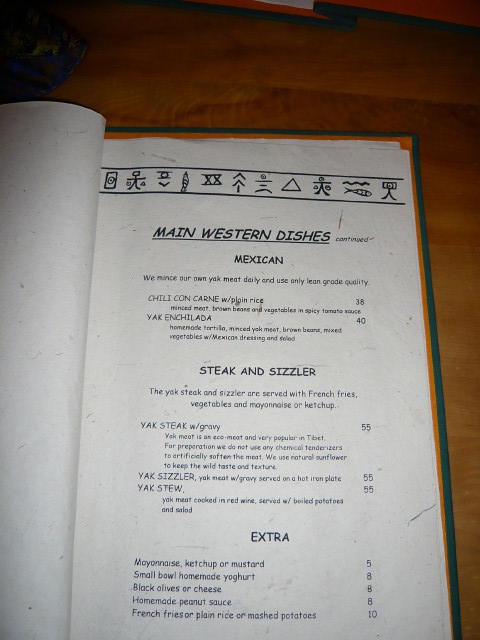Photograph of an open menu resting on a wood-colored table, presented in a book format with the left page folded back. The menu features text in black, highlighted with horizontal black lines at the top, enclosing hieroglyphic-like characters. 

At the top of the visible page, bold lettering reads "Main Western Dishes," which is underlined and followed by smaller text. Directly below, the section "Mexican" is specified, introducing an intriguing note in a smaller font: "We Mince Our Own Yak Meat Daily and Use Only Lean Grade Quality."

The first dish listed is "Chili Con Carne with Plain Rice," priced at 38, described as containing minced meat, brown beans, and vegetables in a spicy tomato sauce. The next offering is "Yak Enchilada with Homemade Tortilla," featuring minced yak meat, brown beans, mixed vegetables, and Mexican dressing. 

Further down, the menu continues with "Steak and Sizzler" sections that list various yak-related items. An "Extras" section is indicated below.